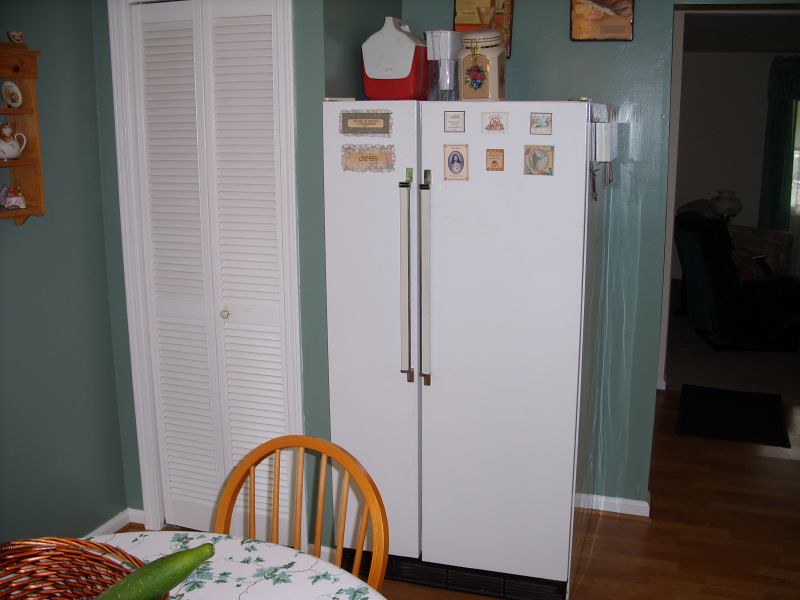This photo, taken inside a house, captures a section of the kitchen with a prominent blue-colored wall and a white, wooden-paneled pantry door. Against the blue wall, a wooden decoration hangs, adding a warm, rustic touch. In the center of the image stands a white refrigerator with two doors adorned with various magnets – two rectangular ones on the left door and six smaller square ones on the right. Above the fridge, a red and white cooler, several containers, and a jar are visible. A few photos partially peek out from behind these items on top of the fridge. In front of the refrigerator, a small table covered in a white cloth with a floral pattern holds a woven basket with a green cucumber inside. Next to the table is a brown wooden chair. The hardwood floor extends through the kitchen, enhancing the cozy ambiance. In the background, on the right side of the image, there is a doorway leading into a living room, where a blue Lazy Boy chair is visible.